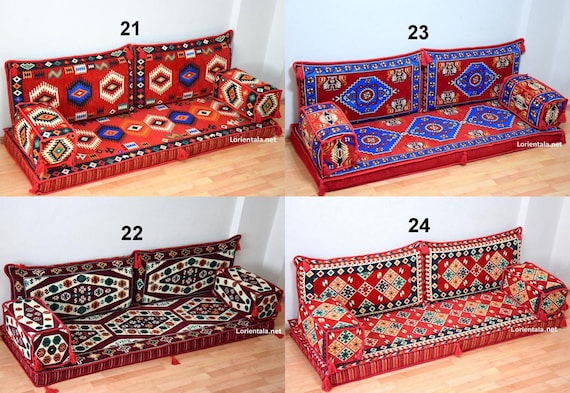The image consists of four photographs, arranged in a two-by-two grid, depicting detailed representations of a unique type of sofa. Each photo showcases a low-lying sofa with a thin mattress directly on the floor, supported by two large back cushions and rectangular armrests, all covered in the same fabric. The photographs emphasize the different fabrics used for each sofa, which are primarily shades of red with varied patterns and accents.

In the top left, labeled "21", the sofa features a Native American-style fabric with reds, blues, and intricate patterns including squares and eye motifs. Below it, labeled "22", the fabric shifts to deep purple hues with whites and touches of green in the patterns. The top right sofa, numbered "23", blends brick red and blue tones with rich, darker blues and indigo hues. The bottom right sofa, labeled "24", is adorned with lighter red fabrics, decorated with yellow squares, triangles, and white stars.

A black number, corresponding to each sofa's label, is positioned above each photo: "21" and "23" at the top, and "22" and "24" at the bottom. A subtle white text or stamp that reads "Lorientals" is faintly visible, potentially signifying a brand or collection. The background of each photo is consistent, featuring a wood floor and a white wall, emphasizing the product focus of the images.